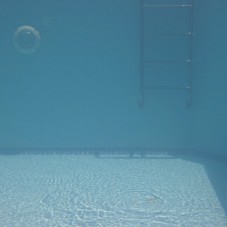This small, low-resolution underwater photograph captures the tranquil and serene environment of an in-ground swimming pool. The water is a clear, luminous blue, with a rippled pattern visible on the sunlit pool floor, while the water above remains calm. On the right side of the image, a metal ladder with four visible steps stretches from the bottom of the photograph upwards, creating a striking reflection on the pool floor. To the left of the ladder, a circular object, possibly a pool light or vent with a white border, is attached to the pool wall. The wall of the pool is a medium blue, contrasting with the lighter blue of the bottom. The photograph, despite being blurry and pixelated, conveys the serene beauty of the underwater scene illuminated by daylight.